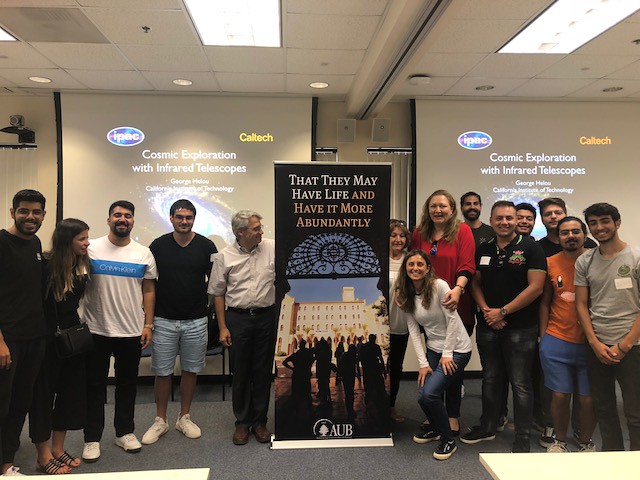In the photograph, taken indoors at a conference or convention under low lighting, a group of around 14 people is gathered in a room. The room features gray carpeting and white hanging tile ceilings with bright white lights. Dominating the center of the gathering is a large rectangular poster with a black background that reads, "That they may have life, and have it more abundantly." Below this text, there's an image of a multi-story building with people dressed up in front of it, possibly denoting Caltech as mentioned in the captions, with "AUB" labeled at the bottom of the image. Surrounding the poster, the group of people, likely a mix of students and a few older individuals, is positioned both to the left and right. On the walls behind them are projector screens displaying texts like "Comic Exploration with Infrared Telescopes," "IPAC," and "Caltech," suggesting a research presentation or career fair context.